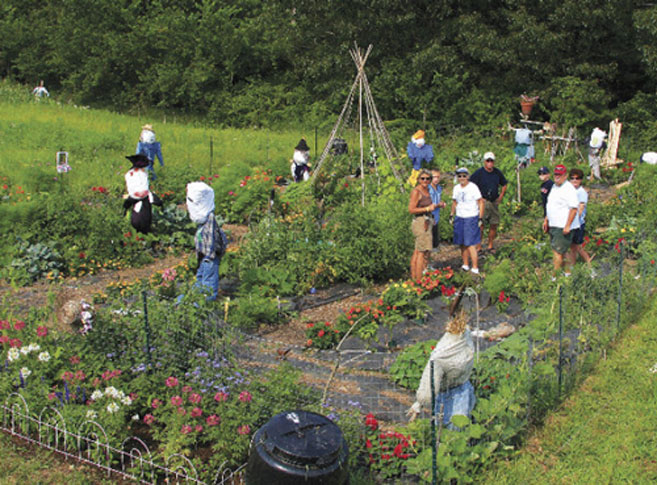The photograph captures a vibrant community garden nestled in a lush, grassy field adjacent to a wooded area with numerous green trees. The garden, rectangular in shape, is bordered by a three-foot-tall metal chicken wire fence supported by thin green posts. At the forefront, there's a smaller arch-shaped fence enclosing a section with white, pink, and blue flowers. Inside the main fenced area, various plants, including orange and red flowers, flourish. 

In the garden's lower left corner, a scarecrow dressed in a plaid shirt with a pillowcase head stands watch, complemented by four additional scarecrows positioned around the perimeter. Central to the scene is a round black tank accompanied by a variety of flowers. A teepee-shaped structure, designed for climbing vines, adds a rustic charm to the garden's layout.

Seven people, donned in casual attire like shorts and t-shirts, are engaged in conversation, contributing to the garden's communal atmosphere. This scene hints at the space being a community garden, inviting individuals from all around to plant and nurture their plots together.